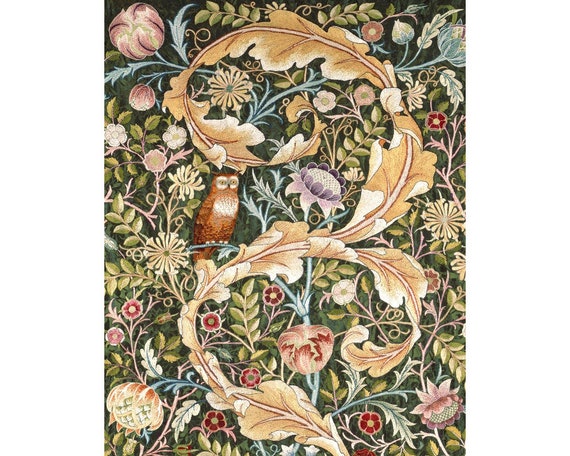This illustration, possibly a detailed wallpaper, shower curtain, or fabric, depicts a highly artistic scene reminiscent of an Alice in Wonderland style. Dominated by a dark green background, it features an intricate array of densely packed foliage and flowers. There are large green leaves and various flowers including muted purple sunflowers, orange blossoms, red flowers, pink velvety flowers, and salmon-colored roses. Some flowers even resemble dandelions in muted yellows and subtle blues. A central feature is a small brown owl with white chest markings and eyes, perched serenely on a branch surrounded by the flourishing flora. The overall palette consists of subdued and harmonious colors, giving the entire piece a whimsical yet tranquil appearance that evokes the charm of a children's book illustration.